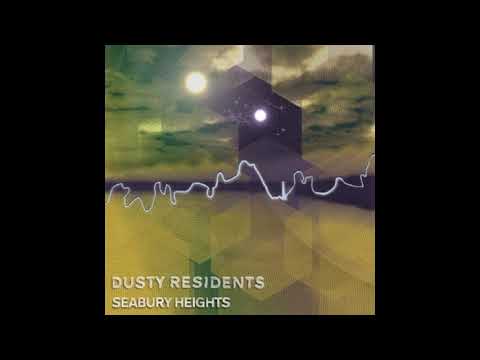The image appears to be an album cover with a thick black border, thicker on the left and right sides than on the top and bottom. Inside the border, the main square is yellowish, filled with cubist and geometric shapes in varying shades of yellow. At the top of the image, there is a faded depiction of a cloudy sky, with the remnants of a skyscraper barely visible. Two sun-like lights add a surreal touch to the upper portion of the artwork. Cutting through the center of the image is a black street overlayed with a wavy white line that adds a dynamic element to the scene. In the bottom left corner of the image, the album title "Dusty Residence" is prominently displayed in white, all caps. Below it, in smaller white caps, is the subtitle "Seabury Heights." The combined elements give the entire piece a modern, abstract feel reminiscent of a unique and thought-provoking album cover.